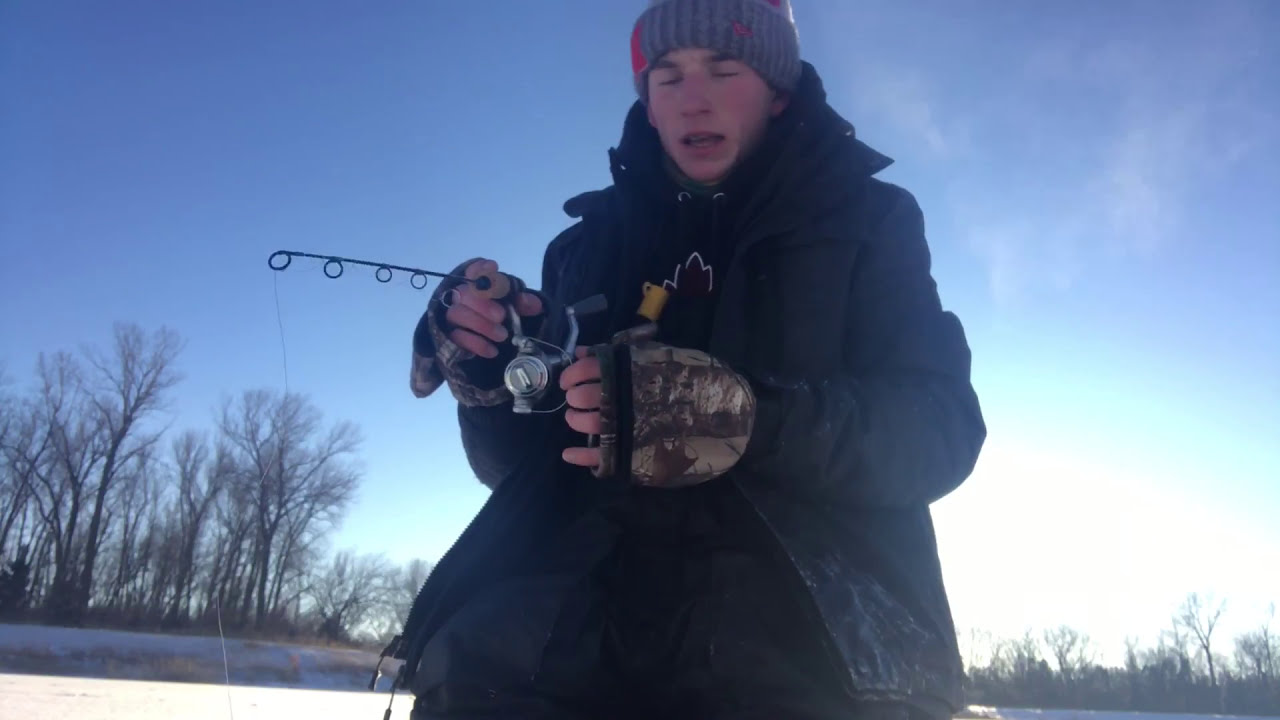In the photograph, a young man, likely in his late teens or early twenties, stands or kneels in a wintry landscape, possibly near a frozen lake. He is clad in heavy winter attire, including a black or dark coat layered over a hoodie, and wears a gray beanie with a red stripe on the left side. His fingers are partly covered by fingerless camouflage gloves, and he holds a modified, very short fishing rod with the line extending directly downward from the reel. The man's eyes are closed and his mouth is slightly open, suggesting a moment of deep concentration or perhaps exhilaration. Behind him, the background features leafless trees stretching up towards the sky, which is a vivid blue with a few wispy clouds on the right side. A snow-covered bank with tufts of light brown grass lies to the left, contributing to the cold, stark ambiance of the scene. A black backpack is also visible in front of him. The camera angle is slightly elevated, capturing an upward view that emphasizes the expansive sky overhead.